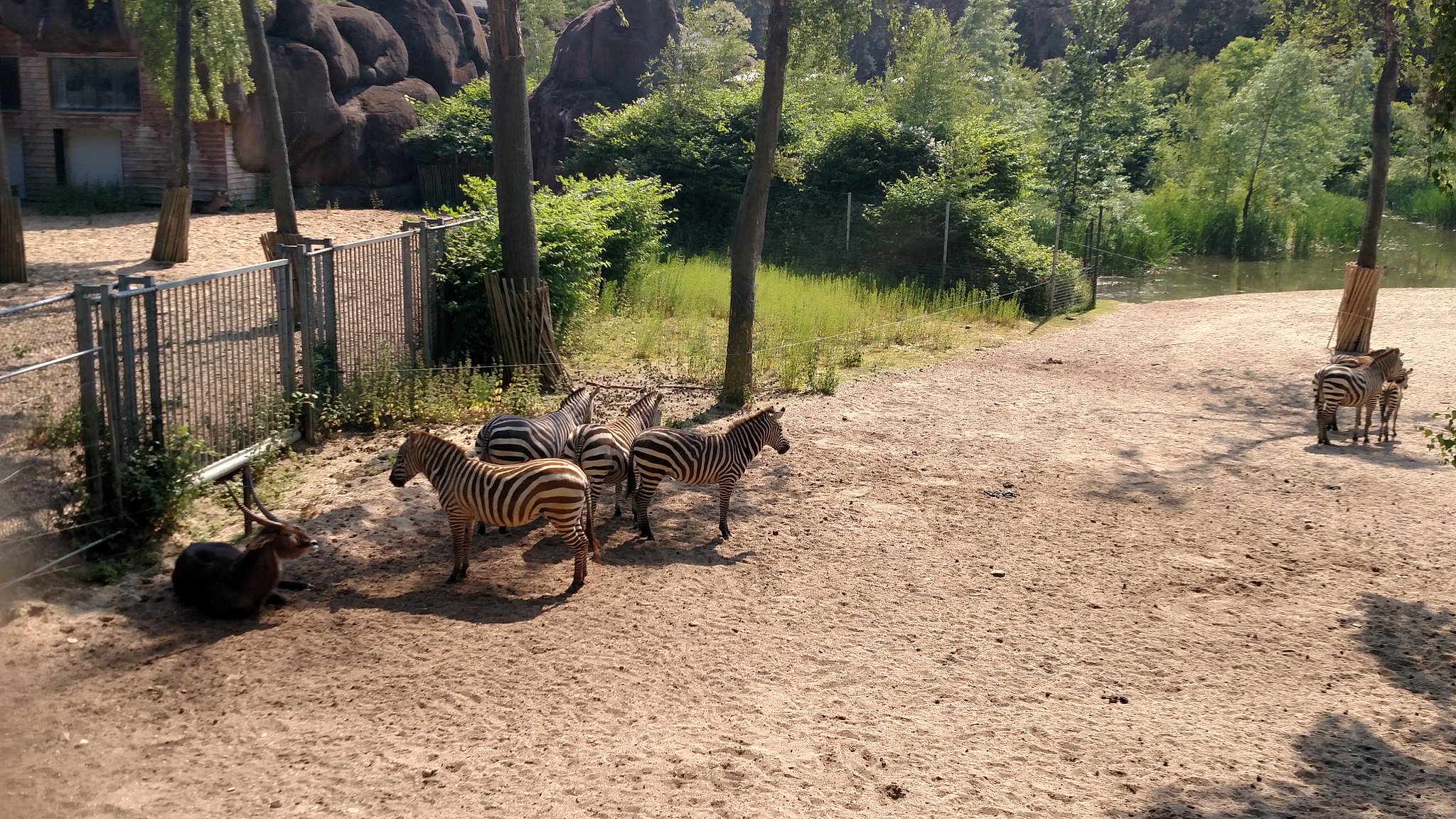The image shows a landscape-oriented, real-life scene likely taken at a nature reserve or zoo, characterized by its fenced enclosure. In the foreground, a sandy, dusty area hosts six zebras—five adult zebras and one baby—spread across the scene. Four zebras are centrally located, with three facing away from the camera and one standing sideways. Two additional zebras are positioned further back near the right edge, gazing off-camera. The setting features mixed greenery in the background, including numerous green trees, small bushes, grass, and some large brown rocks. A hint of a small body of water is visible in the distance. On the left side of the image, a small stone building with cutouts stands partly visible, while a silver fence clearly separates the zebras from this structure and surrounding vegetation. The scene is bathed in sunlight, casting soft shadows and indicating a sunny day with no visible people, suggesting it might be off-hours or simply a lightly attended period. An antelope, dark brown and lying down, is also present on the left, observing the zebras.